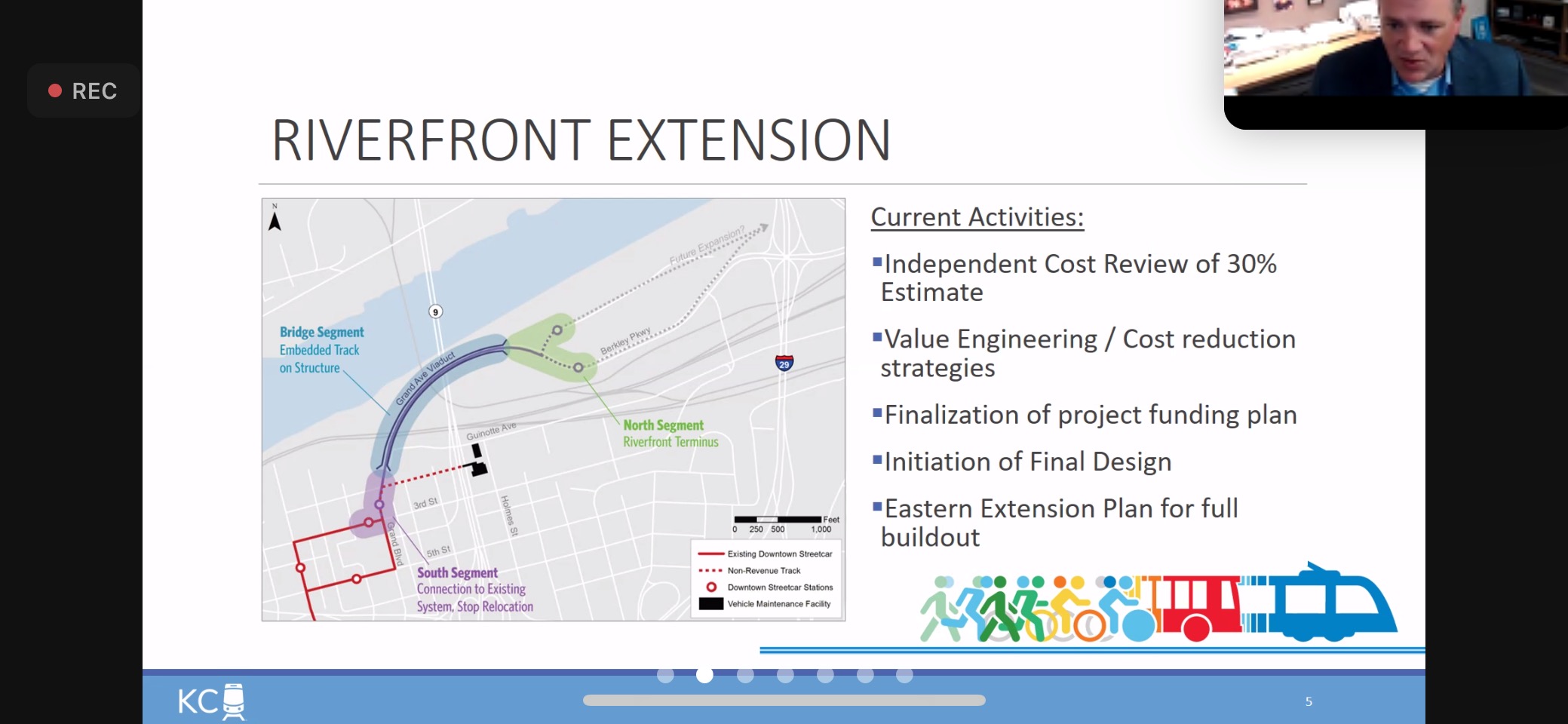The image is a screenshot from a PowerPoint presentation titled "Riverfront Extension," possibly captured during a recording or live stream. The upper right corner of the screen features a small camera view of a man sitting at a desk, looking into his monitor. The recording is indicated by a "REC" symbol with a red dot in the upper left corner. 

The main slide has a white background with black text and colored elements. A prominent feature on the left side of the slide is an overhead view of a map, illustrating a city situated next to a river. This map includes different segments labeled "Bridge Segment," "South Segment," "North Segment," with annotations such as "embedded track on structure," "connection to existing systems," and "riverfront terminus."

At the bottom of the slide, there's a blue navigation bar typical of PowerPoint presentations, showing multiple circular dots that indicate the presentation stage. On the leftmost side of this bar, a logo features the letters "KC," likely representing mass transit, and an emblem in the lower right corner depicts various modes of transportation – from walking and running to cycling, motorcycling, car, bus, and train.

The text on the right side of the slide outlines several project activities:
- "Current Activities"
- "Independent Cost Review of 30% Estimate"
- "Value Engineering/Cost Reduction Strategies"
- "Finalization of Project Funding Plan"
- "Initiation of Final Design"
- "Eastern Extension Plan for Full Buildout"

Overall, the image is clear and vibrant, encapsulating various aspects of the Riverfront Extension project, alongside relevant logistical and developmental details.